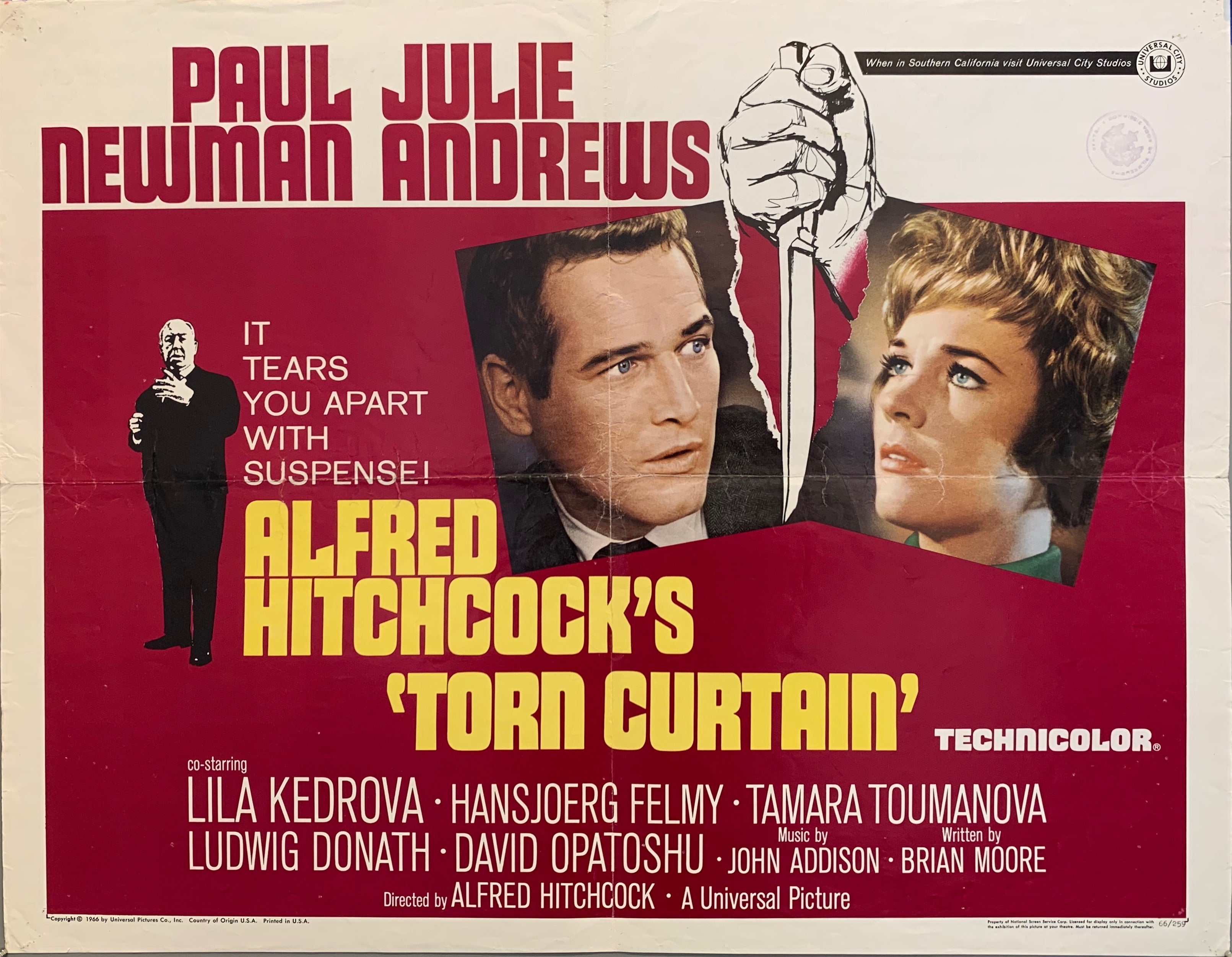The image depicts a vibrant movie poster for the Alfred Hitchcock film "Torn Curtain," featuring Paul Newman and Julie Andrews. The poster's background is a striking red with a gray border. At the top, the names of the leading actors are prominently displayed: Paul Newman and Julie Andrews. Toward the top right, there are dramatic black-and-white photos of Newman and Andrews, torn down the middle by a drawing of a fist clutching a knife. In the middle of the poster, text reads, "It tears you apart with suspense. Alfred Hitchcock, Torn Curtain, Technicolor." To the left, a small image of Alfred Hitchcock stands, adding to the iconic director's signature style. Below this central section, additional cast members are listed: Lila Kedrova, Hans-Jörg Felmy, Tamara Tomanova, Ludwig Donath, and David Opatashu. The production credits note that the movie features music by John Addison, was written by Brian Moore, and directed by Alfred Hitchcock, further establishing its classic suspense thriller atmosphere. The colors present in the poster include yellow, beige, blue, black, white, brown, and the dominant red background, with a visually intricate, suspense-filled design typical of Hitchcock's style.